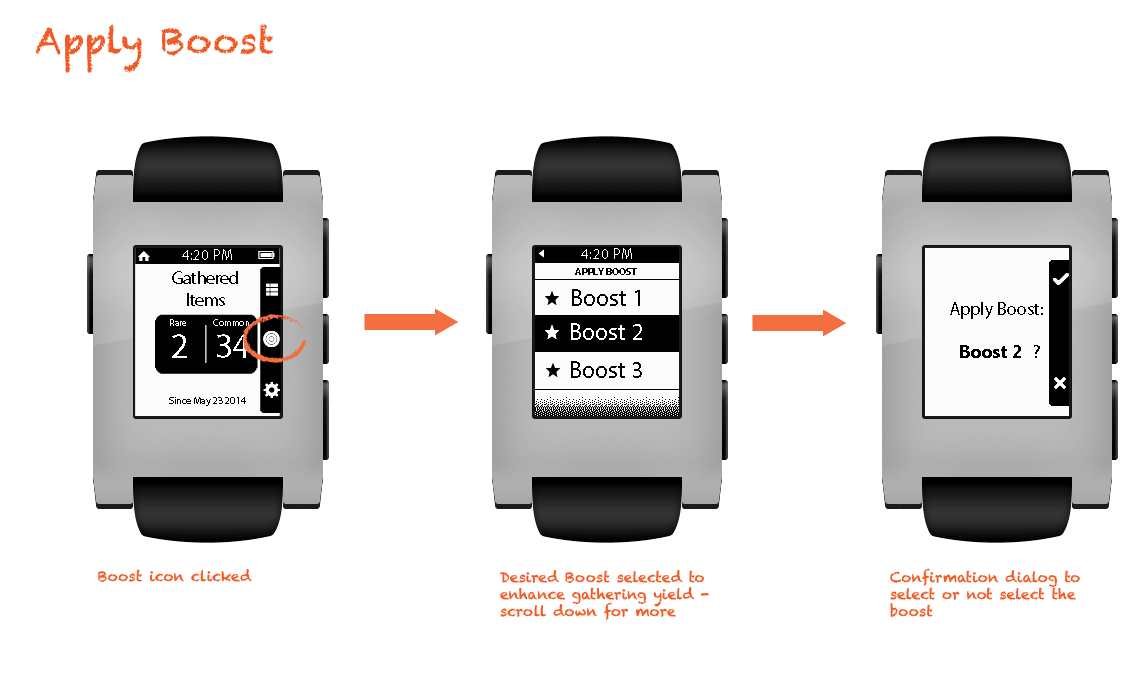The image depicts a detailed diagram with instructions for applying a "Boost" feature on a rectangular, grey and black smartwatch with a black and white screen. The top left corner of the diagram displays the words "Apply Boost." The diagram is divided into three segments, each representing a different screen on the smartwatch. 

1. The first screen shows the time (4:20 PM) along with battery life indicators and has a section labeled "Gathered Items." It includes a house icon and the numbers "2" and "34" displayed within a dark square with a white outline. An icon for the Boost feature is highlighted for selection.
   
2. The second screen provides the option to choose between three boost levels: Boost 1, Boost 2, and Boost 3. An arrow indicates to proceed by selecting the desired boost level, emphasizing Boost 2 as selected, which enhances gathering yield. 

3. The third screen poses a confirmation dialog with the text "Apply Boost 2?" offering a choice between a check mark for confirmation and an X mark for cancellation.

This comprehensive illustration ensures users clearly understand each step to successfully apply a boost on their smartwatch.